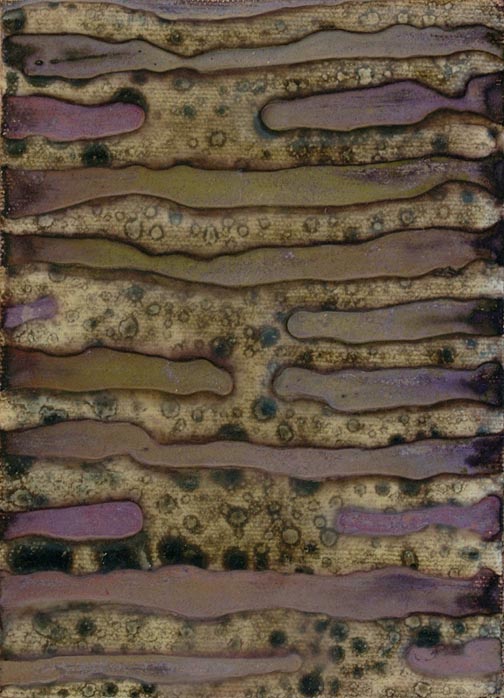The vertically-aligned rectangular image features an intricate, textured background consisting of light brown with a scattered pattern of darker brown outlines and small black-filled circles, predominantly clustered at the bottom left and through the center. Superimposed on this background is a complex maze-like pattern made up of irregularly-shaped, horizontally aligned lines, primarily shaded in varying shades of purple with occasional hints of green. These lines exhibit wavy, almost corpuscular edges that appear to weave in and out of the background, creating the illusion of passing through holes. The sequence of these lines varies, with some stretching fully across the image and others only partway from either side, intermittently interrupted. At the very top, there is a line that spans the entire width, followed by alternating partial and full-length lines beneath. The bottom-most line starts thin on the left and thickens towards the far right. The collective visual effect suggests abstract art, yet also hints at a microscopic or botanical texture, blending organic forms with artistic abstraction.